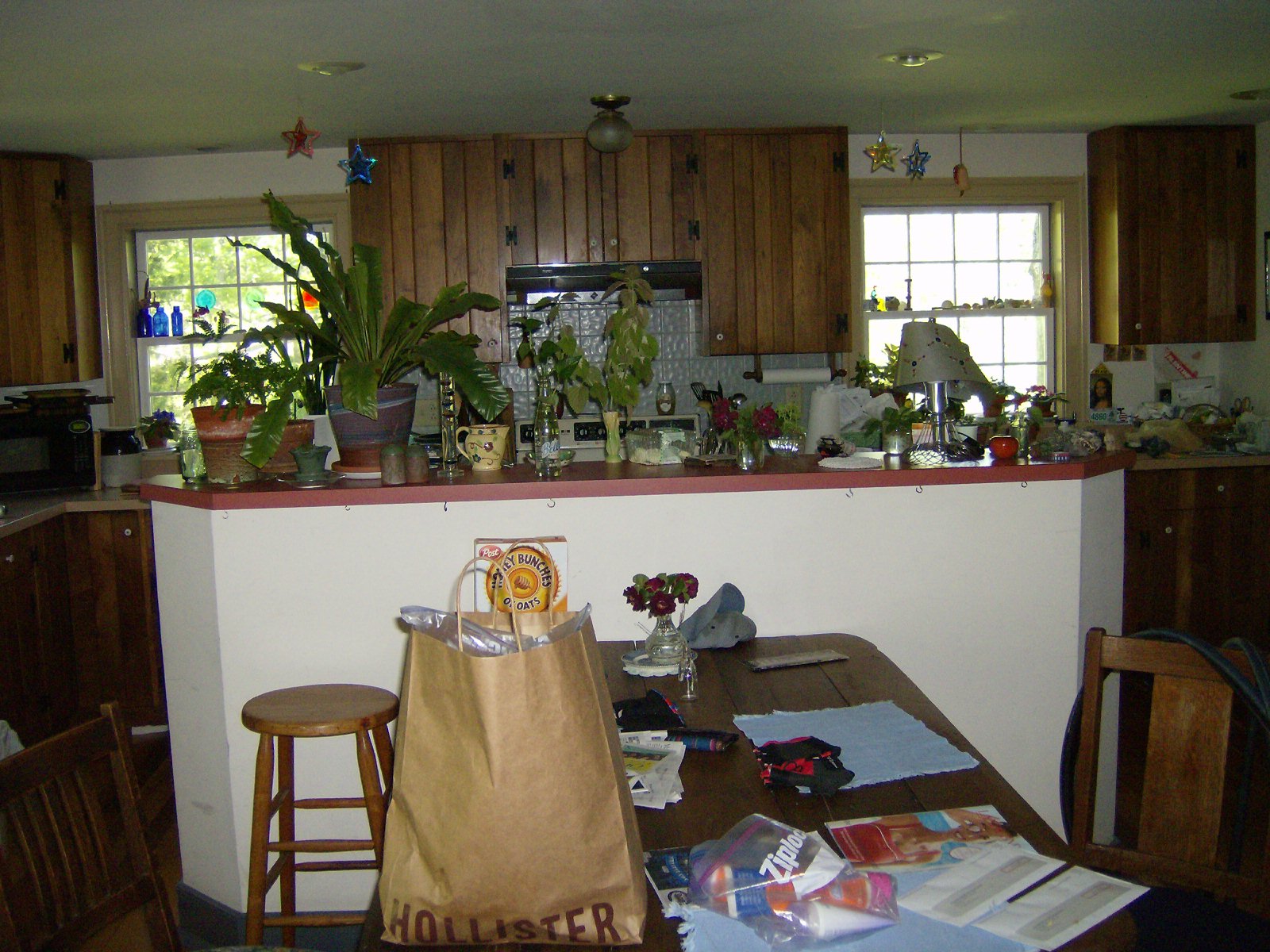A vibrant kitchen space seen from the adjacent dining room, characterized by its homely yet eclectic decor. The long, wooden dining table extends into the foreground, accompanied by two mismatched wooden chairs – one featuring large cutouts on the backrest, and the other with closely stacked wooden slats. To the right, a bar area with a white and red theme supports a singular stool, creating a small, cozy nook.

On the kitchen counter, a brown paper Hollister bag and a Ziploc bag sit amidst a scatter of papers, adding to the lived-in feel. A vase brimming with fresh flowers and a box of Honey Bunches of Oats contribute to the colorful, cluttered arrangement. The large kitchen island, predominately white with red accents, is adorned with a variety of plants, contrasting with the darker paneling of the cupboards towards the back.

Red, white, and blue star decorations dangle from the ceiling, adding a festive touch. Natural light filters through the paneled windows, illuminating the space and highlighting several bottles placed on the window ledges. The kitchen exudes warmth and vibrancy, underscored by a striking silver backsplash that adds a modern flair to the backdrop.